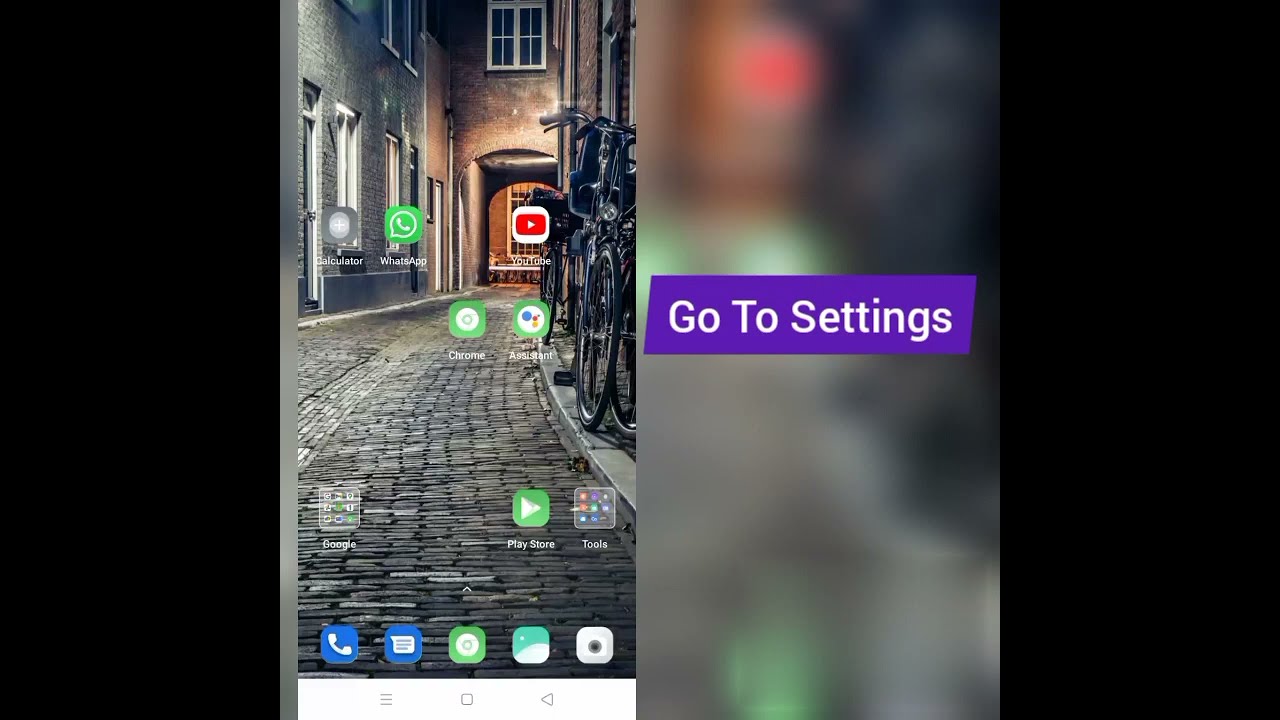This wide rectangular image is divided into four vertical sections. The two outermost sections are the thinnest and are completely black. The central sections illustrate a detailed screenshot of a smartphone’s home screen. The dominant feature of the screenshot is a background image of a picturesque cobblestone pedestrian road leading up to an arched brown brick tunnel. On the left side of the road are gray and brown buildings, while on the right side there is a bicycle rack, giving it a distinctly European feel. Superimposed over this scenic wallpaper are various app icons, including WhatsApp, a calculator, YouTube, Chrome, and the Play Store. At the bottom of the screen, there is a white strip containing five additional icons: phone, messaging, power, weather, and one more icon. Adjacent to this home screen image, on the right section of the screenshot, is a blurry background in shades of black, green, and gray. A purple rectangle with white text reading "Go to settings" is prominently displayed here, enhancing the instructional feel of the snapshot. This composite image suggests a tech-related guide or tutorial involving a smartphone interface.